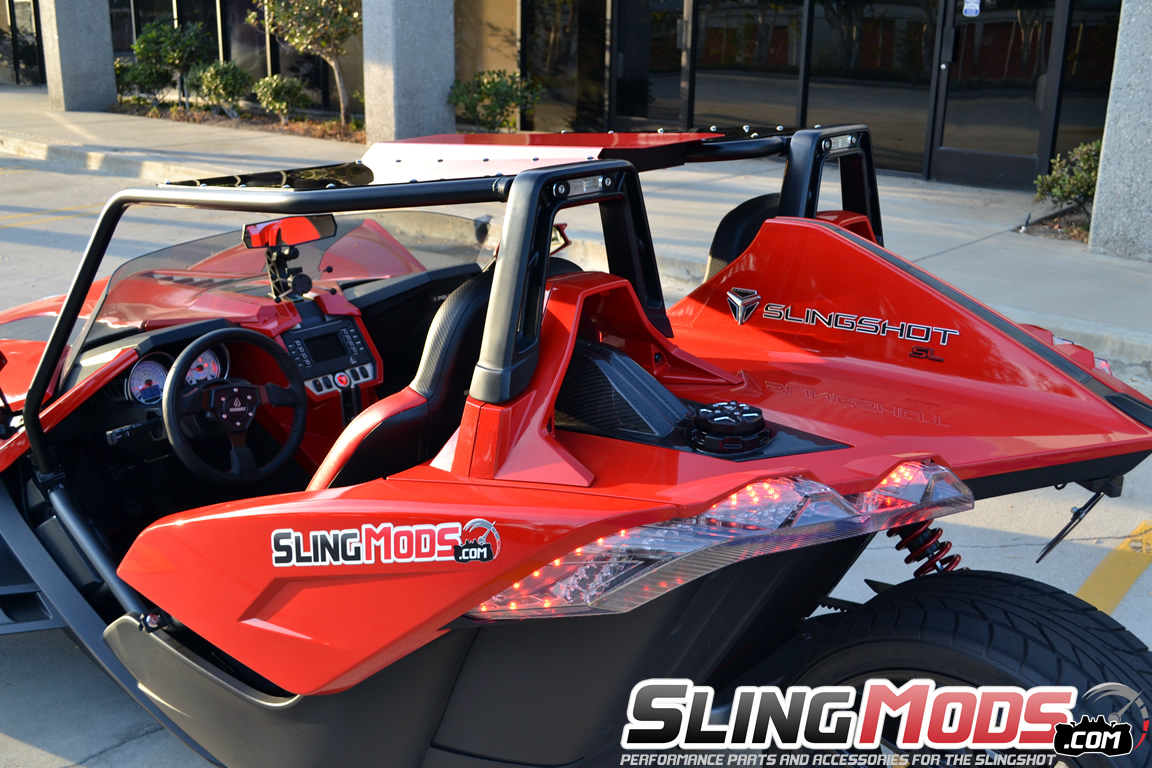This image captures a red and black three-wheeled vehicle, specifically a car-motorcycle hybrid. Known for its sporty appearance, the vehicle features a small, smoky gray windshield that reaches about halfway up its front, which doesn't cover the entire cockpit area. The steering wheel is situated on the left side, offering a clear view of the instrument panel and a central console with a screen. Above the open top is a black roll cage providing a sense of structure and safety.

Emblazoned on the side of the vehicle is the logo "Sling Mods," along with the website address slingmods.com, indicating that it's associated with performance parts and accessories for the SlingShot. The bright red body contrasts with its black detailing, such as visible shock springs and tires. The rear end showcases taillights that appear as small red dots. The unique build consists of one rear wheel and two front wheels, hinting at its three-wheeled design.

In the background, a sidewalk and the glass door entrance of an office building are visible, suggesting the vehicle is parked outside in a populated area. The overall impression is of a high-performance, futuristic vehicle, intended for excitement and style.